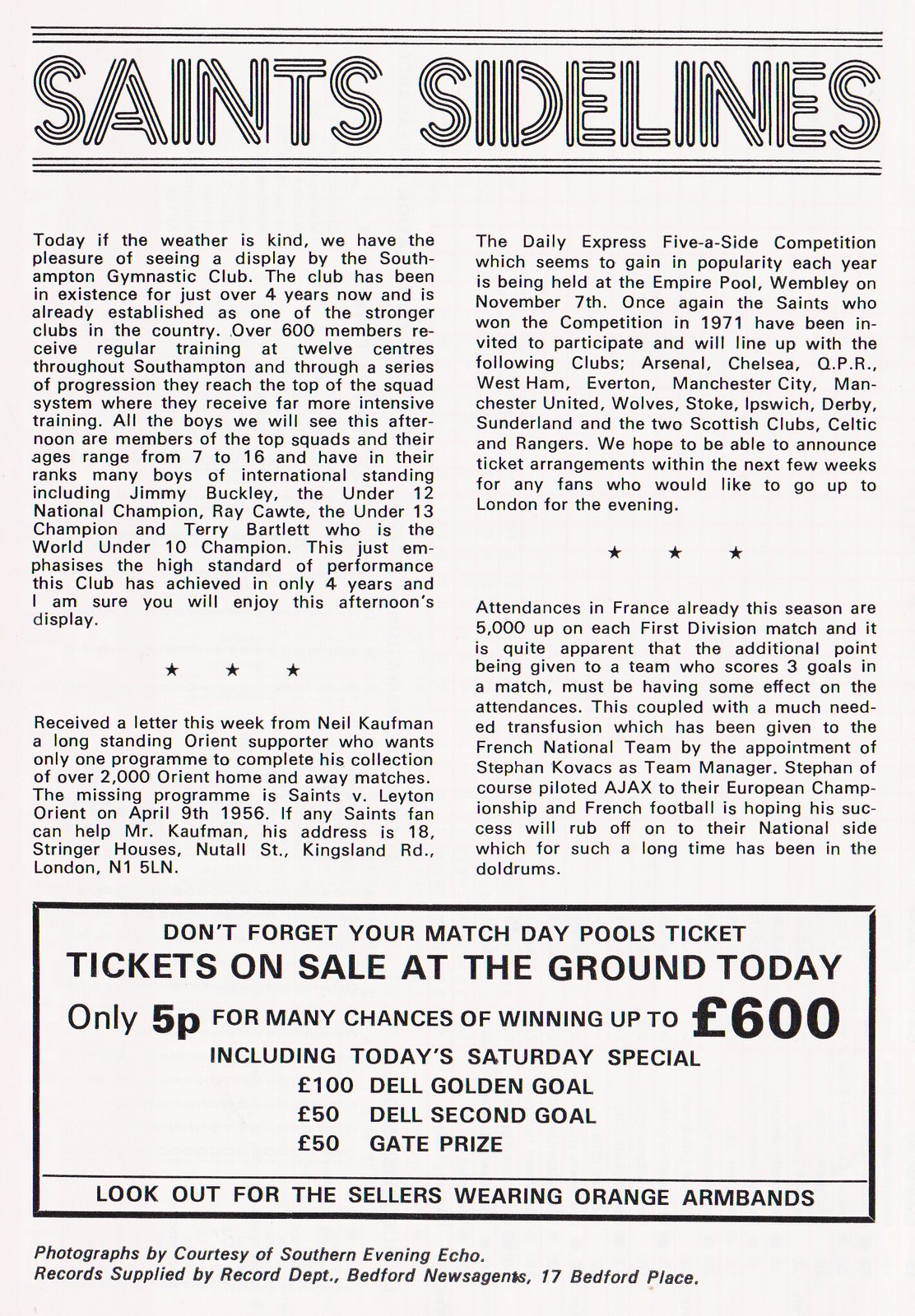This image appears to be a scan of a page, likely from a magazine or newspaper, specifically featuring an advertisement that combines information about the Saints Sideline and instructions for purchasing match day tickets. The top of the page prominently displays the title "Saints Sideline" in a quirky font where the 'S' appears as if it's made out of three spaghetti noodles. Below the title, a detailed article describes a display by the Southampton Gymnastic Club, mentioning its establishment over four years ago and its status as one of the strongest clubs in the country. The text highlights that over 600 members train regularly across 12 centers in Southampton and the province, and it outlines that more intensive training is provided at the top of the squad system.

The article is formatted in multiple paragraphs, with decorative stars separating some sections. At the bottom of the page, a prominent black rectangle advises readers not to forget to purchase their match day pools tickets, which are on sale at the ground for only five pence. The advertisement entices readers with the chance to win up to £600, featuring specific prizes such as the £100 Dell Golden Goal, £50 Dell Second Goal, and a £50 Gate Prize. It also instructs readers to look for sellers wearing orange armbands. The page credits photographs to the Southern Evening Echo and mentions that records are supplied by the Record Department, Bedford Newsagents, with a slightly distorted mention of "17 Bedford Place". The advertisement uses a simple black and white color scheme and occupies the entire image, giving the feel of a comprehensive poster.